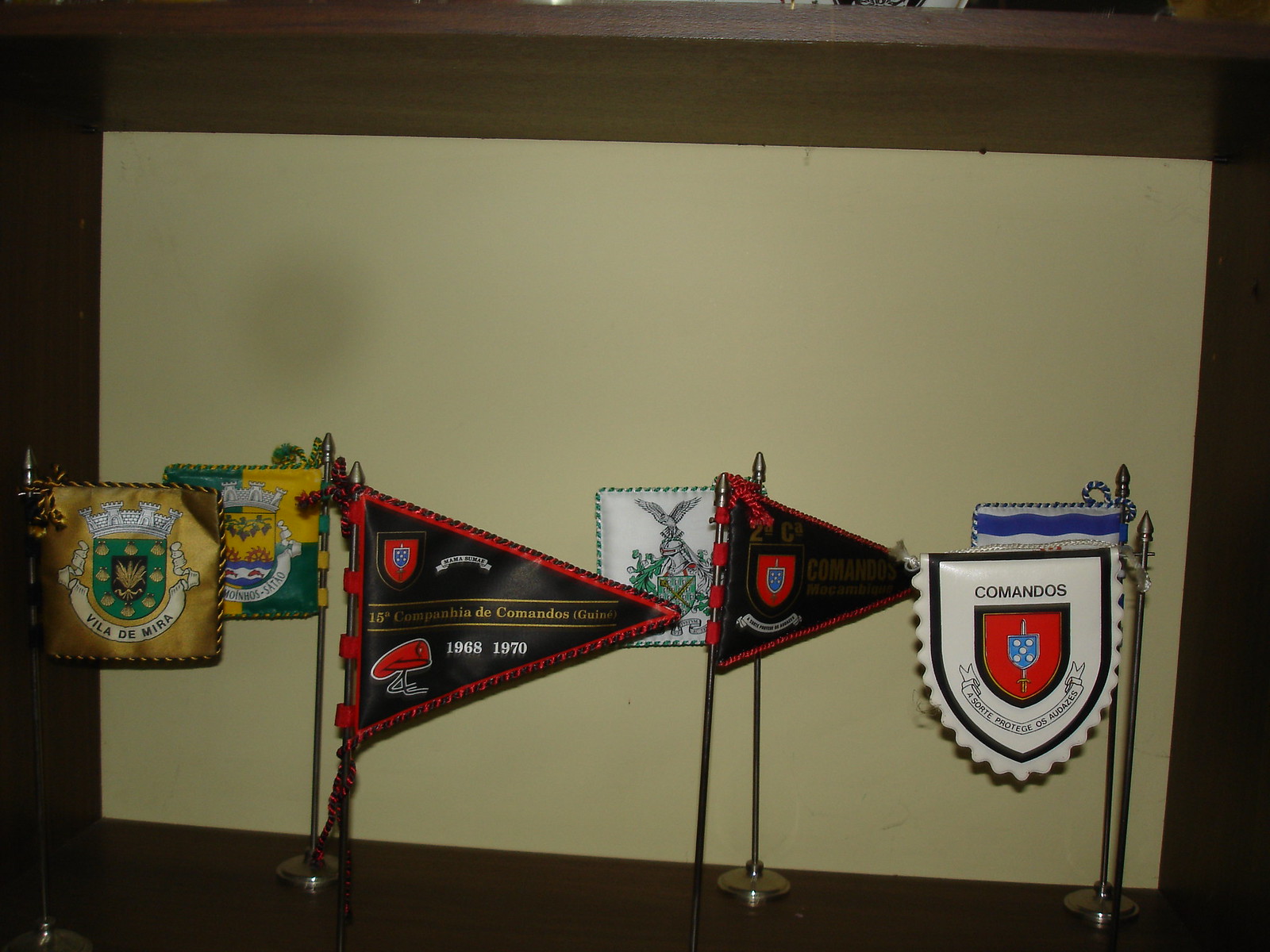This color landscape photograph captures a display cabinet situated in a building, showcasing six distinct commemorative flags, each mounted on small silver or gold poles. The wooden case has a beige background that highlights the diverse flags, varying in size and color. Most flags carry a military theme and incorporate Spanish text. 

One prominent flag is gold and reads "Villa de Mira." Another striking flag behind it is green and yellow, though its text is less discernible. A black triangular flag with red trim stands out, bearing the inscription "15 Compañía de Comandos, 1968-1970." There is a similar triangular flag, partially obscured and difficult to read. Additionally, a white flag prominently displays the word "Comandos." The collection also includes a square flag with gold details and more inscriptions in Spanish, broadening the militaristic and historical significance of the display.